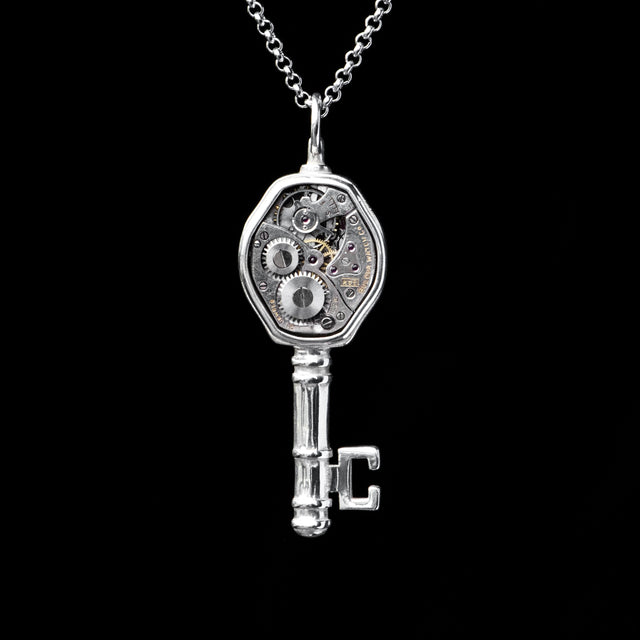The image features a key-shaped pendant on a thin silver necklace, set against a completely black background. The chain is visible at the top of the image, leading down to the center where the pendant is prominently displayed. The pendant itself resembles an antique skeleton key, but with a unique twist: the key's bow and barrel are intricately filled with tiny gears, screws, and mechanisms, reminiscent of the inner workings of a watch. This steampunk-inspired design gives the key a clockwork appearance without actually functioning as a timepiece. The pendant exudes a handcrafted, homemade charm, suggesting it might have originated from a crafts market or an online platform like Etsy. The overall effect is both vintage and whimsical.